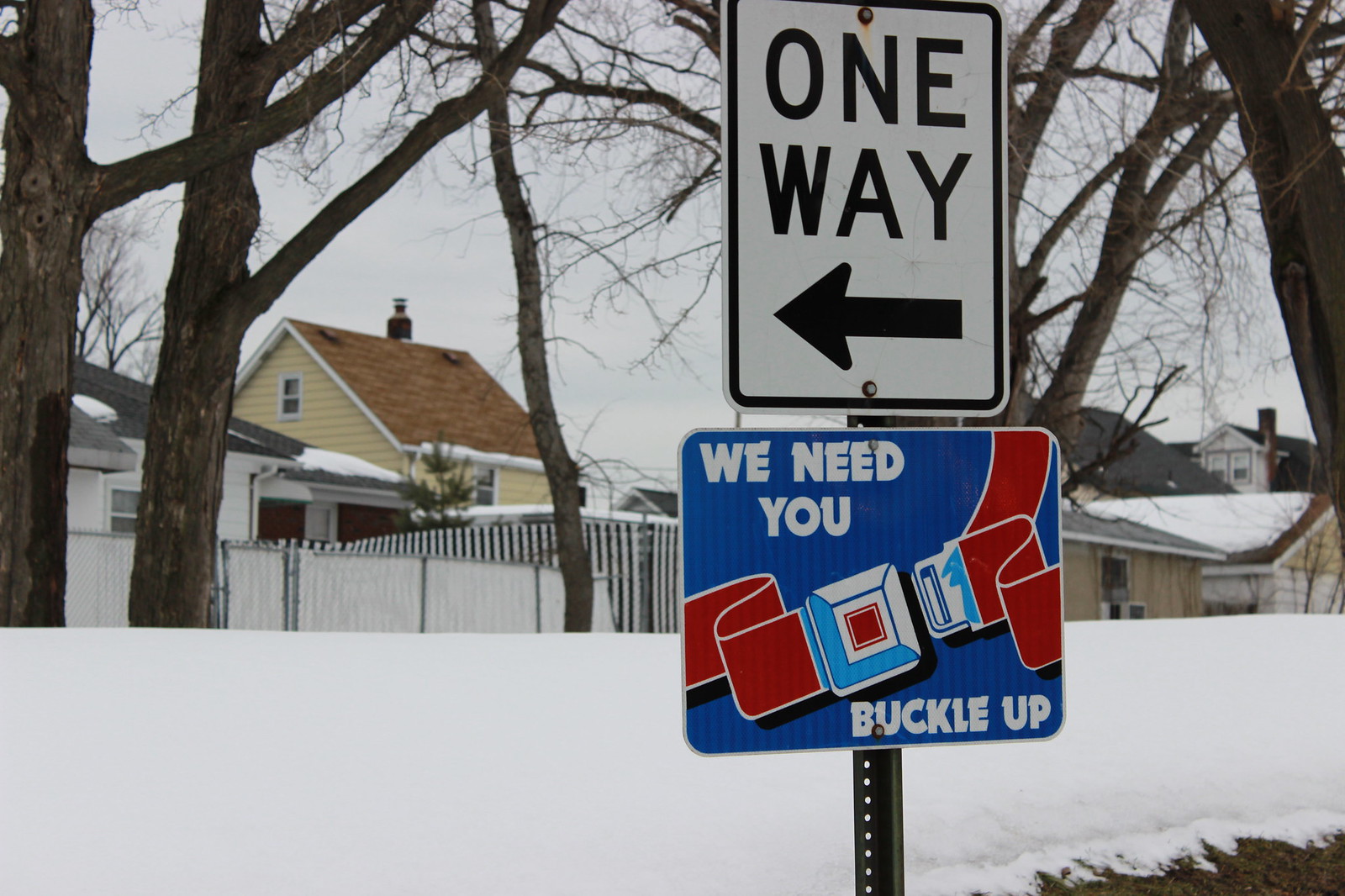In this daytime, overcast photograph likely taken on a winter's day, we see a snowy outdoor scene featuring two prominent road signs in the foreground, slightly right of center. The top sign is a standard U.S. "One Way" street sign with a white background and black trim, bearing black lettering and an arrow pointing to the left. Below it is a blue rectangular sign with a graphic of a seatbelt being buckled, accompanied by white text that reads "We Need You" at the top left and "Buckle Up" on either side of the graphic. The background is dominated by a mound of pure white snow, three tall tree trunks to the left, and another tree trunk to the right. Behind these trees, we glimpse two-story homes, including a yellow house with brown steeply pitched roofing left of center. The image is well-lit and captures the intended public service announcement to encourage seatbelt use against a wintery backdrop.